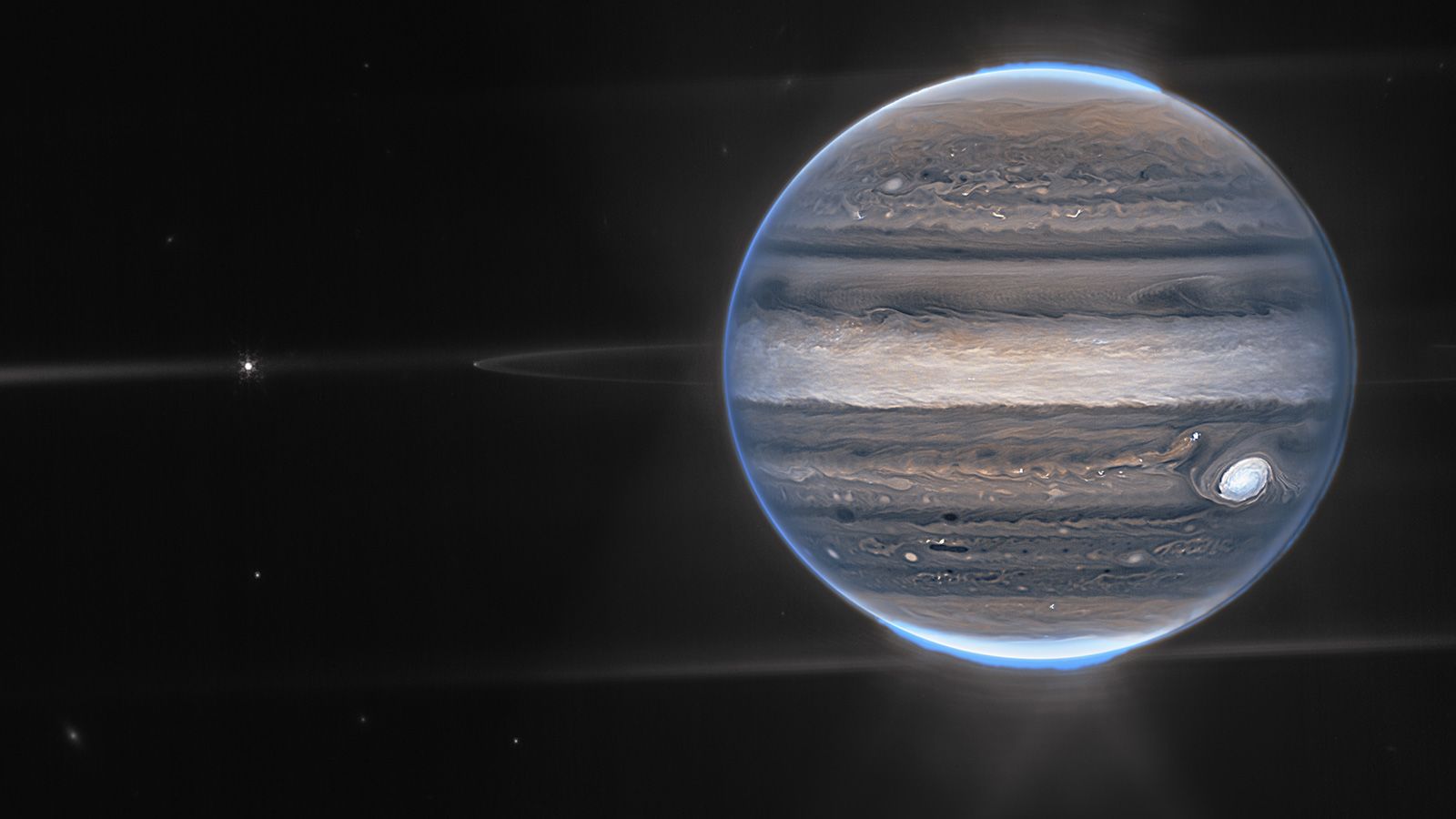This detailed image, potentially a photograph or an exceptionally detailed drawing, captures a surreal depiction of outer space. The background is solid black, dotted with small white specks representing stars, one of which is particularly pronounced on the middle left side, radiating faint lines. Dominating the right side of the horizontally aligned rectangular image is a detailed planet with a striking and complex appearance. 

The planet is encircled by a faint blue and purplish glow, highlighting its spherical shape. The surface of the planet features distinctive horizontal bands of varying colors and textures. The topmost band is a bumpy grayish-brown, transitioning into a smoother brown area, followed by a tan-colored section in the center. The bottom part returns to brownish hues with additional gray tones. A white streak, resembling a swirl, is visible just below the middle white band and adjacent gray area.

Additional details include a light emanating from the planet, creating a soft glow around its edges, particularly on the bottom and top, with less intensity on the right side. Along the bottom edge of the planet, a faint white line stretches from the left of the image, arcs beneath the planet, and continues off to the right. A similar faint line extends from the middle towards the right side, forming a dot and a light ring around the planet. The image, containing no text or context, captivates with its rich detail and ethereal quality, leaving the viewer to ponder its origin and the identity of the depicted planet.